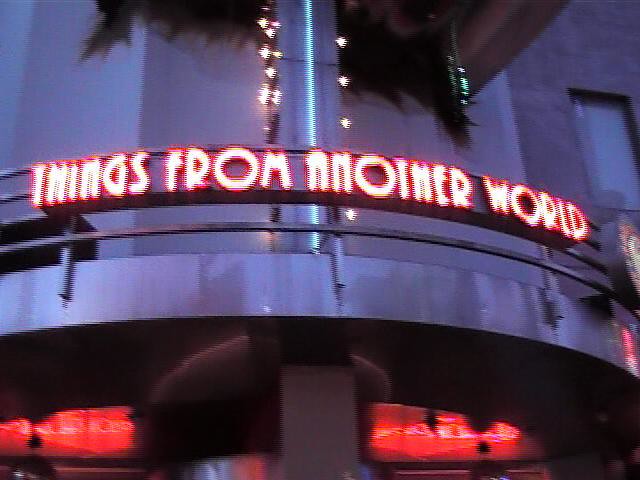The image depicts the exterior of a building that likely serves as a movie theater or stage area, prominently featuring the sign "Things from Another World" in glowing red neon letters. A dark gray, metal-framed structure supports the sign, which has a row of yellow lights along its sides. Above the sign, brown, fluffy decorations that resemble feathers or wings adorn the building. The upper right corner showcases a window framed by the grayish wall. At street level, two sets of red lights illuminate the entrance area, adding vibrant color to the scene amidst the overall dark gray exterior. Beneath the neon sign, there is a thin line of blue neon, and a separate red and gold symbol adds additional detail on the right side. The photo, slightly blurry, is taken outside and captures the urban ambiance, hinting that this location is likely in a large city.